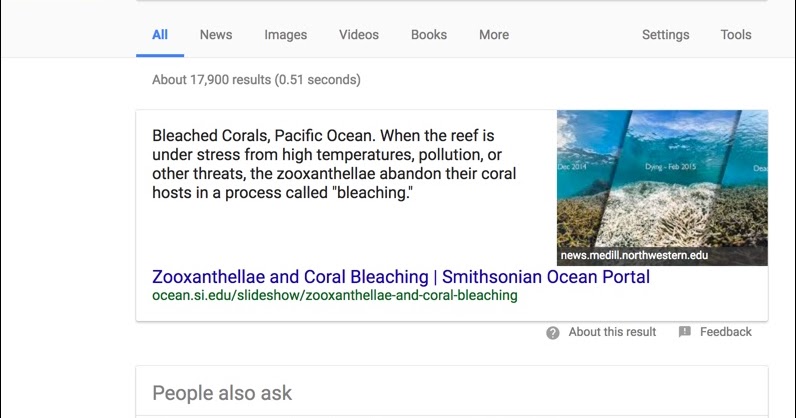This image is a landscape-oriented screenshot of a Google search results page. In the upper left corner, it shows the Google logo and menu options such as "All," "News," "Images," "Videos," "Books," "More," "Settings," and "Tools," all underlined. Although the search query is not visible, the results returned indicate approximately 17,900 hits.

On the right side of the page, there is an image sourced from Northwestern University. The image depicts coral bleaching in the Pacific Ocean, where stressed corals expel their symbiotic algae, zooxanthellae, due to high temperatures, pollution, or other threats. The left side of the image shows healthy coral in December 2014, while the right side illustrates the bleached and dying coral just two months later, in February 2015. This comparison highlights the rapid deterioration of coral within a short time period. 

The text accompanying the image includes an explanation of coral bleaching from the Smithsonian Ocean Portal, emphasizing the devastating impact of environmental stressors on coral reefs. The image is part of a slideshow from ocean.si.edu.